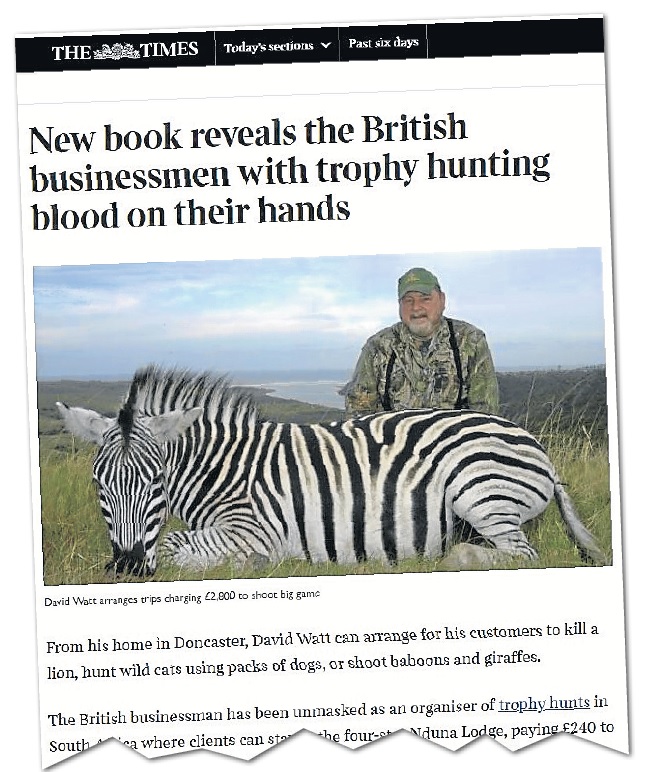This detailed caption provides a comprehensive description of a notable screenshot captured from The Times website:

In this screenshot from The Times, we see the online news website's interface. The top left corner prominently displays The Times' logo. Adjacent to it on the right is a clickable section labeled "Today's Sections," offering various content categories. Further to the right, there is another clickable section titled "Past Six Days."

Beneath these navigational elements, a headline reads: "New book reveals the British businessman with trophy hunting blood on their hands." Accompanying the article is an image of a man dressed in a camouflage shirt and green hat. He sports a dark gray beard and appears slightly overweight. The man is also wearing suspenders and is seated in front of a black and white zebra, giving the impression that he may have hunted the animal.

The caption below the picture identifies the man as David Watt and states: "David Watt arranges trips charging £2,800 to shoot big game." The text continues, noting that from his home in Doncaster, David Watt offers clients the opportunity to hunt a lion, chase wild cats with packs of dogs, or shoot baboons and giraffes.

The article further reveals that the British businessman has been exposed as an organizer of trophy hunts in South Africa. Unfortunately, the remaining text is cut off and difficult to read, making the full extent of the information unclear.